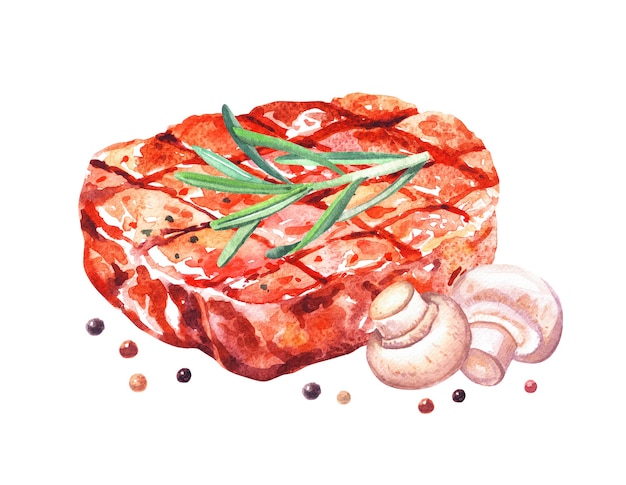This artwork, possibly created with watercolor or colored pencils, depicts a large, thick piece of meat in rich, marbled reds that suggest a combination of raw and cooked elements. The steak features an intricate square grill pattern, with darker red lines crisscrossing its bright red surface, indicating it has been grilled. Atop the steak, a fresh sprig of green thyme rests centrally, extending about halfway across the meat. To the right, two brown mushrooms are touching the meat: one is upside down with its stem pointing upwards, while the other lies on its side with the stem angled towards the ground. Surrounding these main elements are scattered dots in shades of brown, red, tan, and black, resembling unground pepper rounds or assorted spices, adding a vibrant and textured detail to the composition.